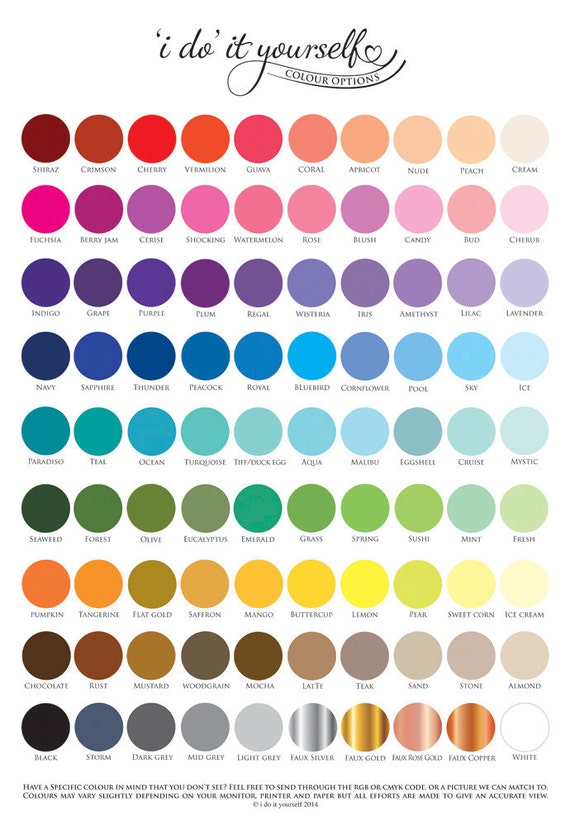The image displays a series of circular paint samples, organized in gradients from darker to lighter shades. At the very top, the title "I do it yourself" is prominently featured in cursive, along with a curving line that states "color options." There are 12 rows of colors exhibited on a white background. The first row transitions from a very dark red, almost brown, to a light cream. The next one starts with fuchsia and lightens to a very light pink. Following this, a gradient moves from indigo to lavender. The subsequent row goes from navy to a lighter shade. Other rows feature gradients from turquoise, dark green, orange, to various browns, and finally from black to white. Every color sample is labeled individually with text underneath each dot, and additional small-sized text appears at the bottom, though it is hard to decipher.